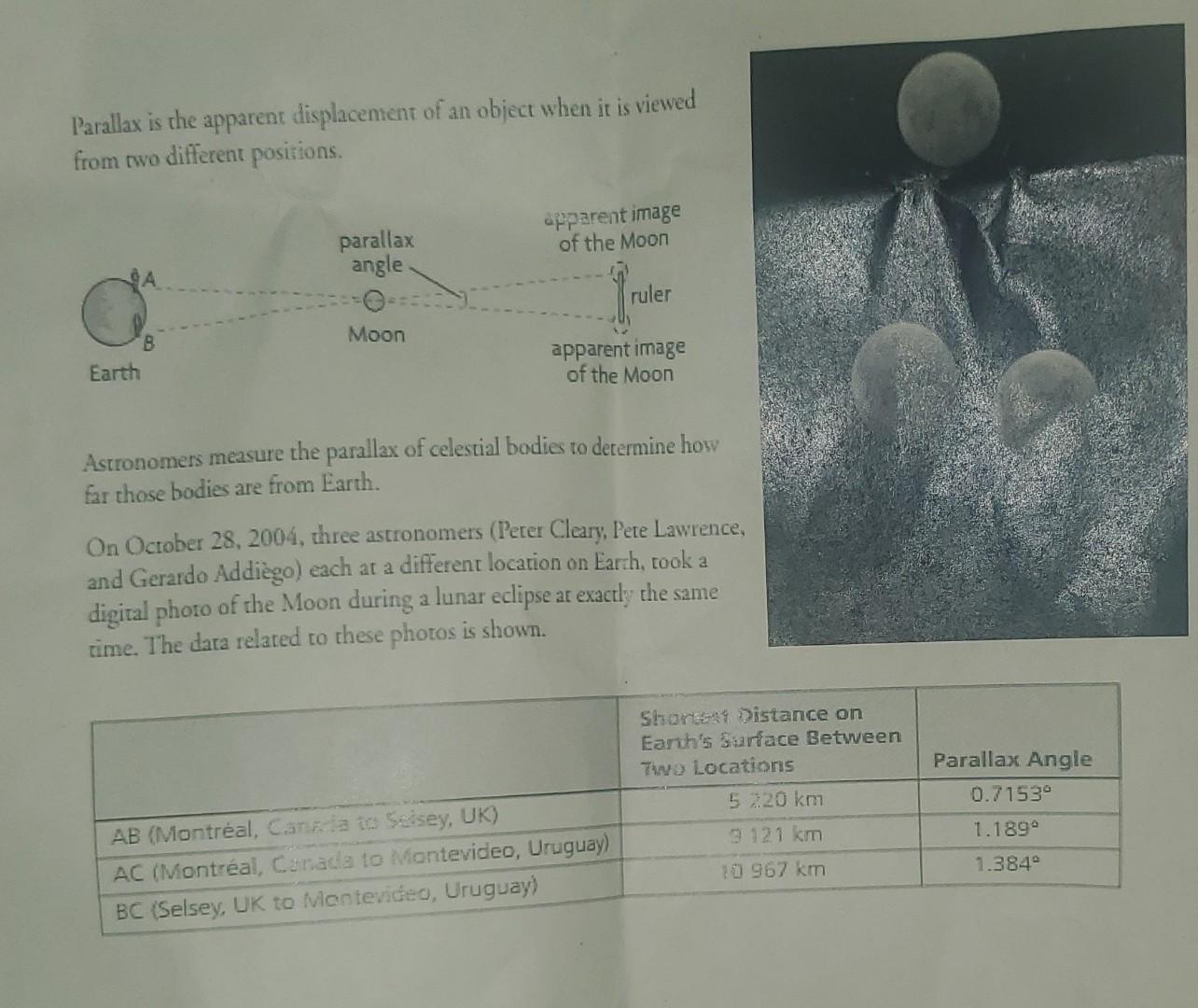The black and white image appears to be a page from a textbook or school worksheet focused on astronomy, detailing how to measure the parallax angle of the moon from Earth. The text explains that parallax is the apparent displacement of an object when viewed from two different positions. A diagram accompanies this, showing the Earth and the moon, with indications of the parallax angle and the apparent image of the moon from two different viewpoints. Additional text notes that astronomers on Earth, including Peter Cleary, Pete Lawrence, and Geraldo Adego, took synchronous digital photos of the moon during a lunar eclipse on October 28, 2004, from different locations. At the bottom of the page, a table presents detailed data: the shortest distances on Earth's surface between Montreal, Canada, Celsius, UK, and Montevideo, Uruguay, and their corresponding parallax angles. For instance, the distance from Montreal to Celsius is 5,720 kilometers with a parallax angle of 0.7153 inches; from Montreal to Montevideo is 9,121 kilometers with a parallax angle of 1.189 inches; and from Celsius to Montevideo is 10,967 kilometers with a parallax angle of 1.384 inches.